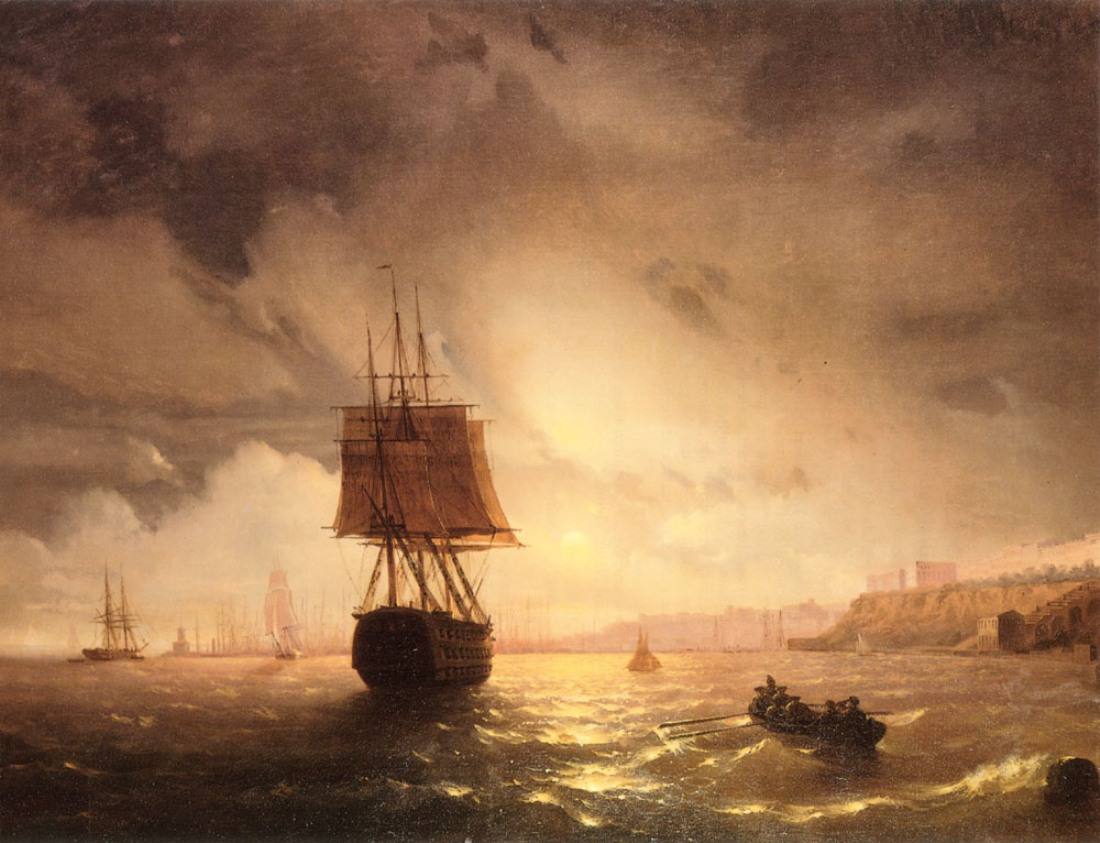The painting showcases a vintage, wooden sailboat with prominent tan-brown sails at its center, slightly left of the midpoint, set against a dramatic sky that transitions from dark, foreboding clouds with eerie yellow tinges to a brighter backdrop. The canvas, predominantly rendered in amber, gray, and gold tones, captures a choppy sea with light reflecting off gentle waves. To the right, a filled rowboat manned by several oarsmen makes its way towards the sailboat. In the lower right-hand corner, a cliffside with fading structures is visible, and several blurred ships dot the distant horizon. The overall composition evokes a sense of movement and impending storm, enhancing the vintage maritime atmosphere.